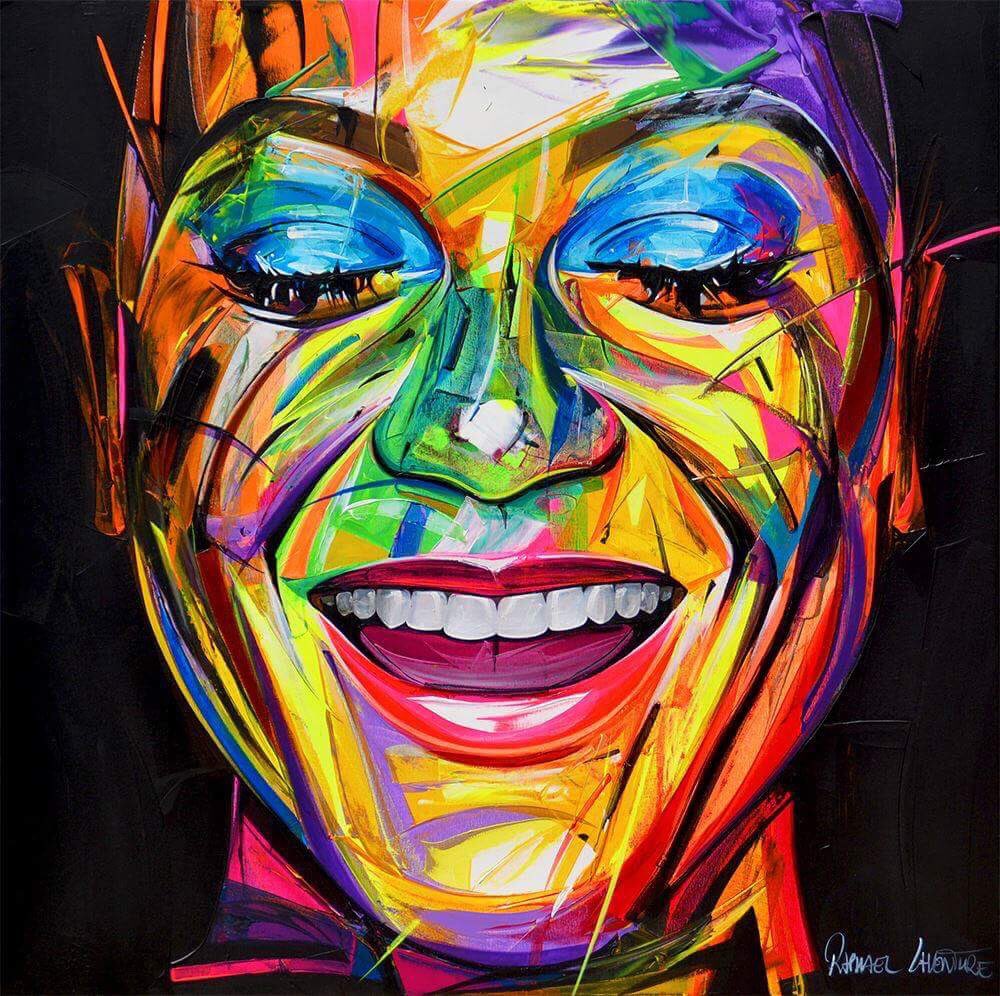This square canvas features a vividly abstract painting of a woman's face, rendered in an array of bright, diverse colors that span the entire rainbow. The background is stark black, which enhances the vividness of the hues used for the face. The face appears from the forehead down to slightly below the chin, without any visible hair or neck background details. Her facial features possess a remarkable volume and are distinctly separated by color segments: her forehead is divided into orange, white, and purple sections, the nose has a greenish tint, and her cheeks transition from orange on the left to yellow on the right. 

Her eye shadow is a striking bright blue, matching the thick mascara strokes above her closed eyes. The red lips are slightly parted, revealing her teeth and a dark pink tongue, giving an impression of a subtle smile. The neck underneath is divided into pink on the left side and orange on the right. 

The background features faint line details and subtle swirls that frame the face subtly. A signature is faintly visible in white in the bottom right corner of the painting, though it remains unreadable. Overall, the painting utilizes a vibrant color palette with sections of bright yellows, greens, blues, reds, and pinks, creating a mesmerizing and abstract portrayal of the woman's face.